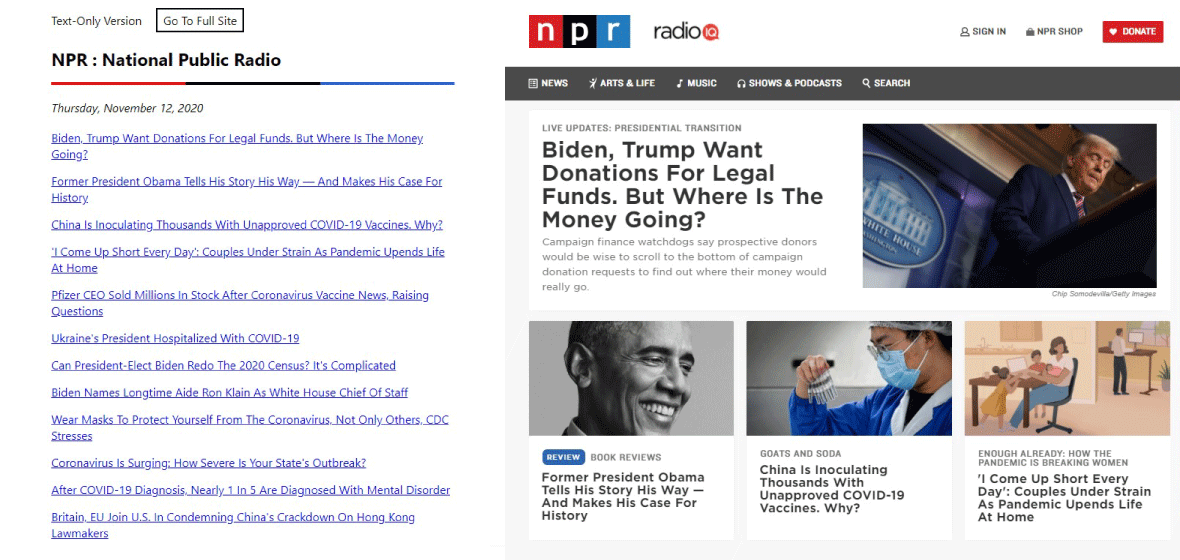An NPR article titled "Presidential Transition" features a prominent black header that includes tabs for News, Arts & Life, Music, Shows & Podcasts, alongside a search bar and live updates. The main headline reads: "Biden, Trump Want Donations for Legal Funds, But Where is the Money Going?" The article advises potential donors to carefully read the fine print at the bottom of campaign donation requests to understand the true allocation of their contributions. Additional stories highlighted include Former President Obama recounting his personal narrative and perspective on historical events, China administering thousands of unapproved COVID-19 vaccines with no clear explanation, and the severe impact of the pandemic on couples, causing daily strains as life at home is disrupted. Capping the piece is a troubling statistic: nearly 20% of individuals diagnosed with COVID-19 are later diagnosed with a mental disorder. This is all compiled by NPR, the public radio network.